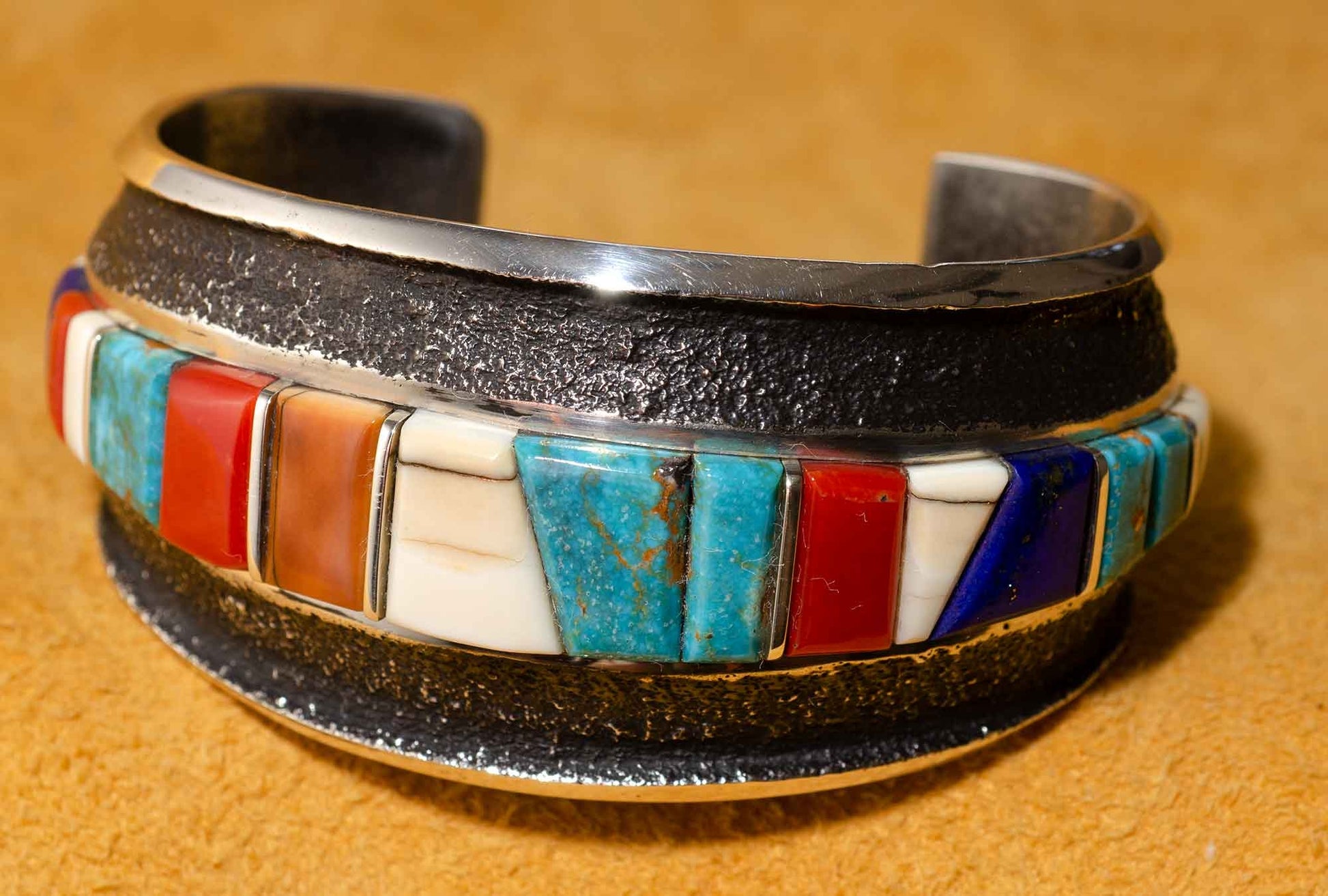This detailed caption is a cleaned-up and enhanced version of the provided description:

"This southwestern-style cuff bracelet features a striking combination of raw and polished silver, crafted into a thick and sturdy accessory. The centerpiece showcases a stunning array of natural, untreated stones including turquoise, fossil ivory, rich red coral, and deep blue lapis lazuli. These stones are meticulously cut into various shapes such as rectangles and diagonal interlocking patterns, creating a dynamic and intricate design. The bracelet rests against a textured mustard-colored background, emphasizing its vibrant colors and exquisite craftsmanship."